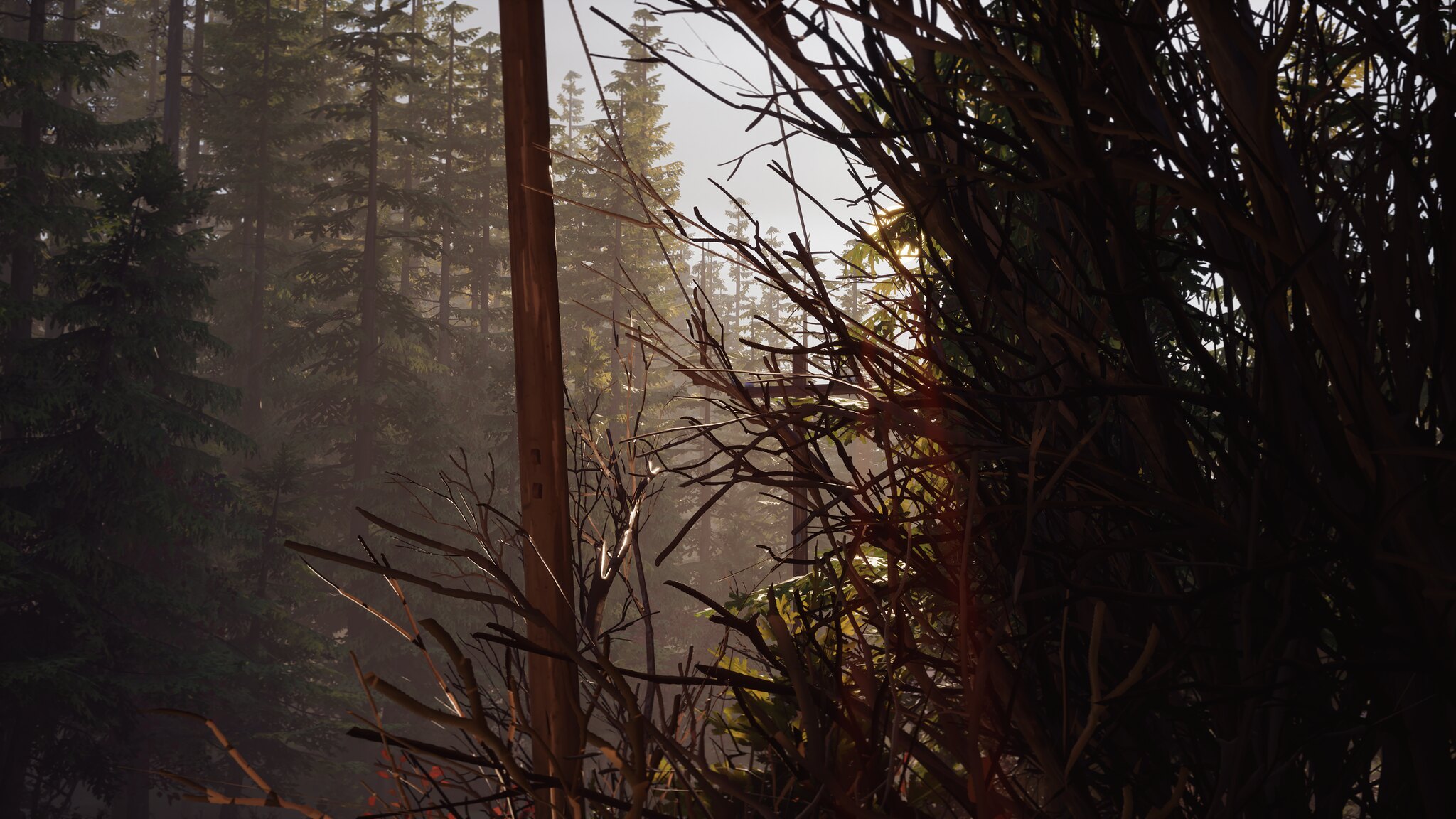The image depicts a dense forest scene with elements that can ambiguously suggest it might be a game screenshot due to the somewhat artificial texture of the vegetation. Occupying the center of the landscape-oriented frame is a prominent brown pole, which could either be a wooden utility pole or a thick tree with a blotchy, somewhat painted appearance. The left side features tall evergreen trees, likely pines, which despite their usual greenery, look exceedingly dry. The right side of the picture is dominated by a shadowed bundle of leafless, dry branches, giving a stark contrast to the otherwise forested area. The background reveals more tall trees, hazily blurred, perhaps by a very early sunrise or a mist, suggesting a naturally lighted but dry forest atmosphere. The absence of any game interface elements adds to the photorealistic quality of the scene.